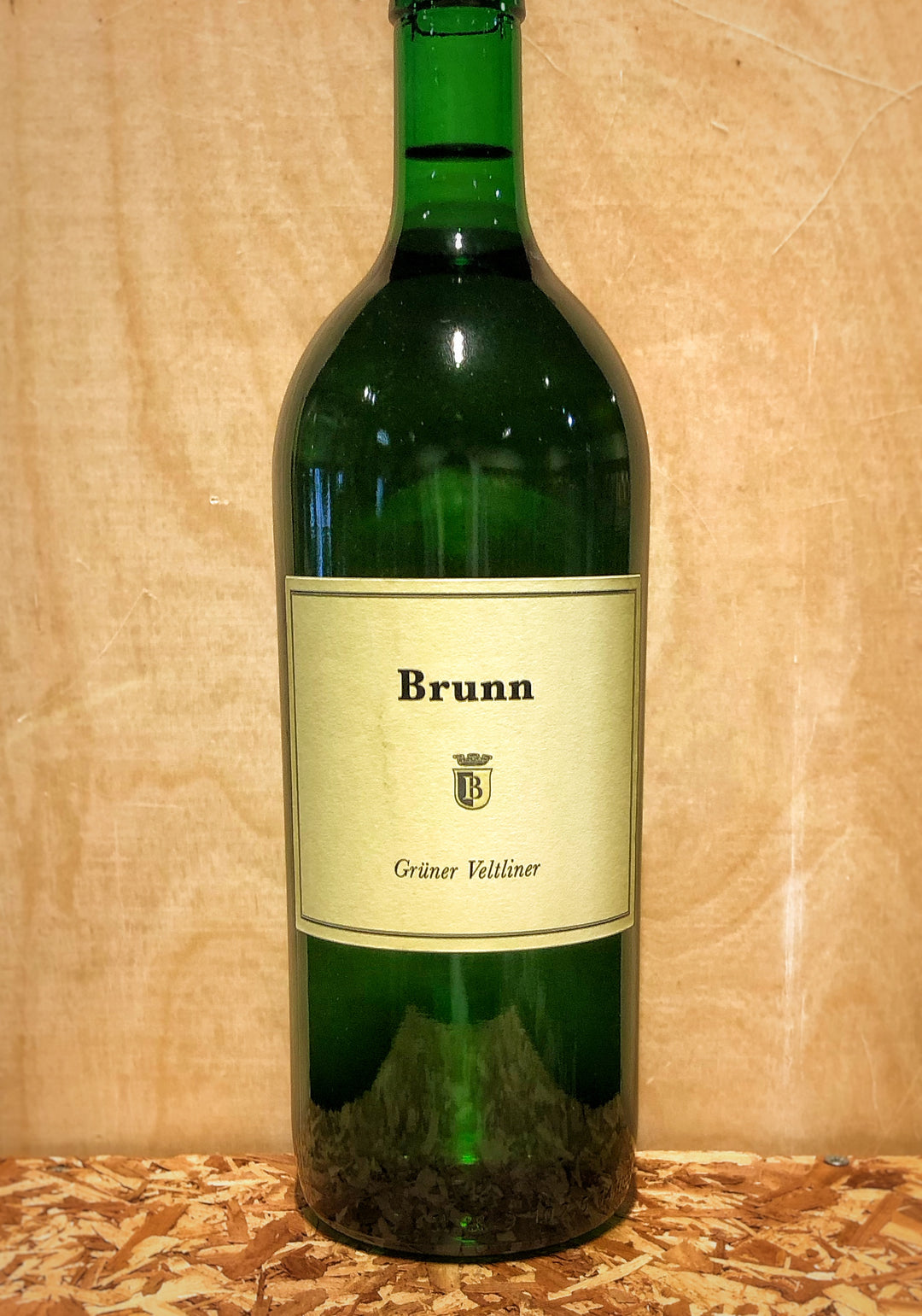This is a portrait-oriented photograph of a green glass bottle seated on a light brown OSB board surface, set against a wood background that appears to be a large plank of light brown wood. The bottle is missing the top part in the image, so the type of cork or screw cap is not visible. The liquid inside appears clear. The bottle features a tan, square label with a thin black border. At the top of the label, bold black text spells out "Brunn" (B-R-U-N-N). Below this, there is a distinctive coat of arms with a crowned shield emblem. The shield is divided vertically with the left half black and the right half white, bearing a prominent letter "B" in alternating white and black colors per side. Underneath the crest, the term "Grüner Veltliner," written in cursive italic font, suggests the type of beverage, though it is unspecified whether it's wine or water.